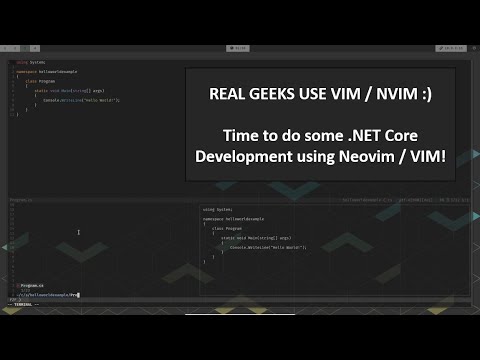A cluttered programming environment in dark mode is displayed, showcasing the text editor Vim, which is popular among programmers for its efficiency. The window is partially obscured, giving it a dim, grayed-out appearance, as another window is overlaid on top of it. The screen is divided into at least three different panes, each containing text that is too small to discern. Horizontal bars are visible at the top and bottom of the image, adding to the complexity. The overall implication is a recommendation for using Vim, or its modern counterpart NeoVim, particularly for .NET Core development, emphasizing its appeal to dedicated, experienced programmers.